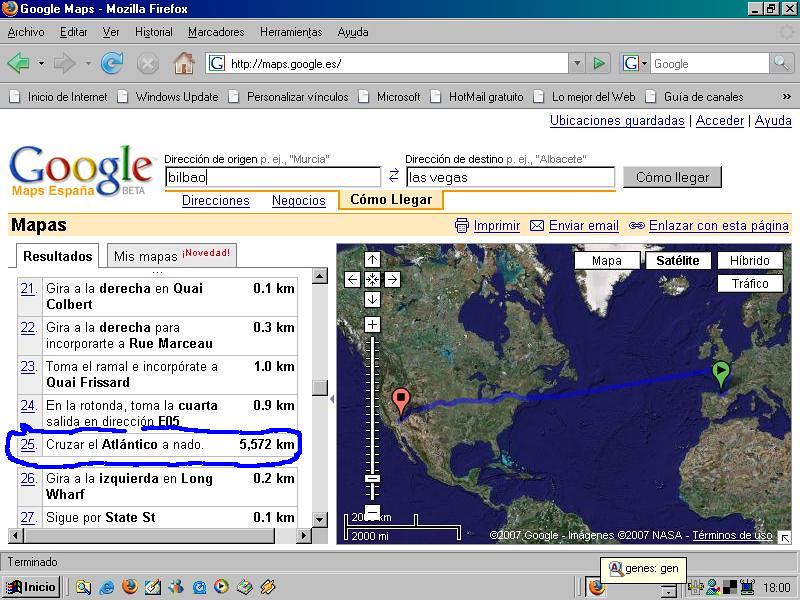The image captures a Google Maps screen displayed in Mozilla Firefox. At the top, there's a blue bar indicating "Google Maps - Mozilla Firefox." Below this, a gray banner provides various browser options. The primary content is in Spanish, with the white Google search bar displaying "Google" and a label indicating "Maps España."

On the left side of the screen, a list of locations marked 21 to 27 is displayed, along with corresponding addresses and distances in kilometers. The central part of the image features a world map showing a travel route. There's a starting point marked with a red pin in Las Vegas, United States, and an endpoint marked with a green dot in Bilibo, located above Africa.

A highlighted blue line traces the route from Las Vegas to Bilibo, covering a total distance of 5,572 kilometers. The map includes specific step-by-step directions in Spanish, detailing turns and road names such as "Gira a la Derecha en Cuy Colbert" and "Toma el ramal a la Incorporate a Cuy Frisard." A notable instruction circled in blue states, "Cruzar el Atlantico a Nado" (Swim across the Atlantic).

The right side of the screen depicts a portion of the map with two landmasses, the United States and Europe, illustrating the transatlantic journey. The screen's bottom features another gray banner with additional options.